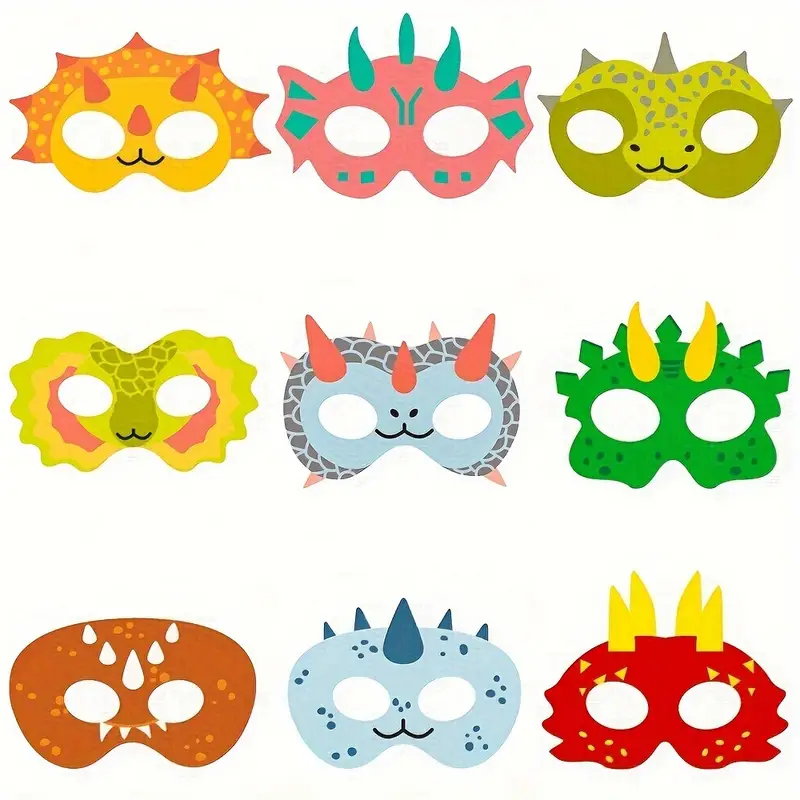The image depicts printable mask templates arranged in a 3x3 grid against an ivory-tinted background. Each mask features vibrant, dinosaur-inspired designs. In the top row, the left mask is yellow with a black mouth, large white eyes, and orange spikes. The middle mask is pink with green horns and turquoise fins on the sides. The right mask is olive green with gray spikes. The second row starts with a mask colored in green, adorned with a pink and yellow crest and green spots. The middle mask in this row is blue with pink horns and gray features. The mask on the right is green with yellow spikes. On the bottom row, the first mask is brown with white horns. The middle mask is blue, decorated with blue dots and blue horns. The final mask in the bottom right corner is red with yellow spikes.